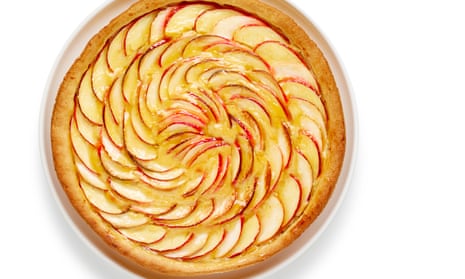In this image, we see a small square culinary photograph featuring a homemade apple tart presented on a white plate. The tart's golden-brown crust extends nearly to the edge of the plate, indicating a perfect bake. The centerpiece of this dessert is arranged meticulously with very thinly sliced apples, fanned out in a striking spiral pattern that starts from the center and winds outward, covering the entire surface. The apples, still adorned with their red peel, lend a vivid red and white contrast to the spirals, enriching the visual appeal. The spiral consists of six concentric circles, with the slices becoming slightly larger towards the outer edge. A yellowish creamy substance can be seen around the apple slices suggesting there might be a subtle sauce or glaze, and the apples appear to be seasoned, possibly with cinnamon, adding an aromatic touch to the presentation. The overall impression is one of a beautifully crafted, appetizing dessert seen from a top-down perspective.